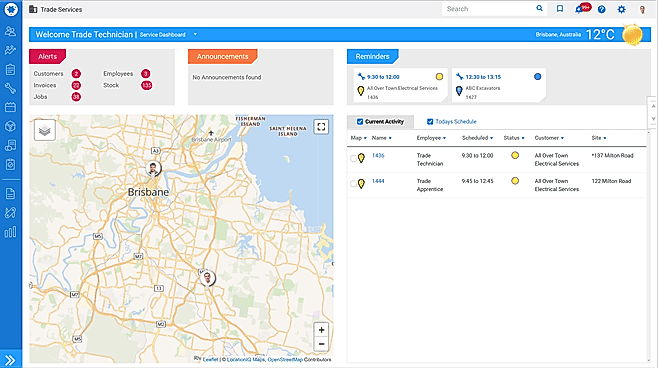This detailed image depicts a user interface of a map-based tool, likely focused on trade and service management, with a location identified as Brisbane, Australia. At the top of the interface, a light gray bar features the title "Trade Services" accompanied by a search box on its right. Adjacent to this bar, there are icons for bookmarking, notifications (with a red bubble showcasing pending alerts), a blue circular question mark for help, a blue gear for settings, and a golden key icon.

Immediately below this top bar, a blue banner warmly welcomes users with the message: "Welcome, Trade Technician Service Dashboard." To the right of this banner, the current weather in Brisbane, Australia is displayed, showing a temperature of 12 degrees Celsius with a sun icon indicating sunny conditions.

Further down the interface, various alerts are organized under categories such as "Customers," "Invoices," "Jobs," "Employees," and "Stock." There are also sections dedicated to "Announcements" and "Reminders." Below these, users can find a detailed "Current Activity" section along with "Today's Schedule," providing a comprehensive overview of ongoing and scheduled tasks.